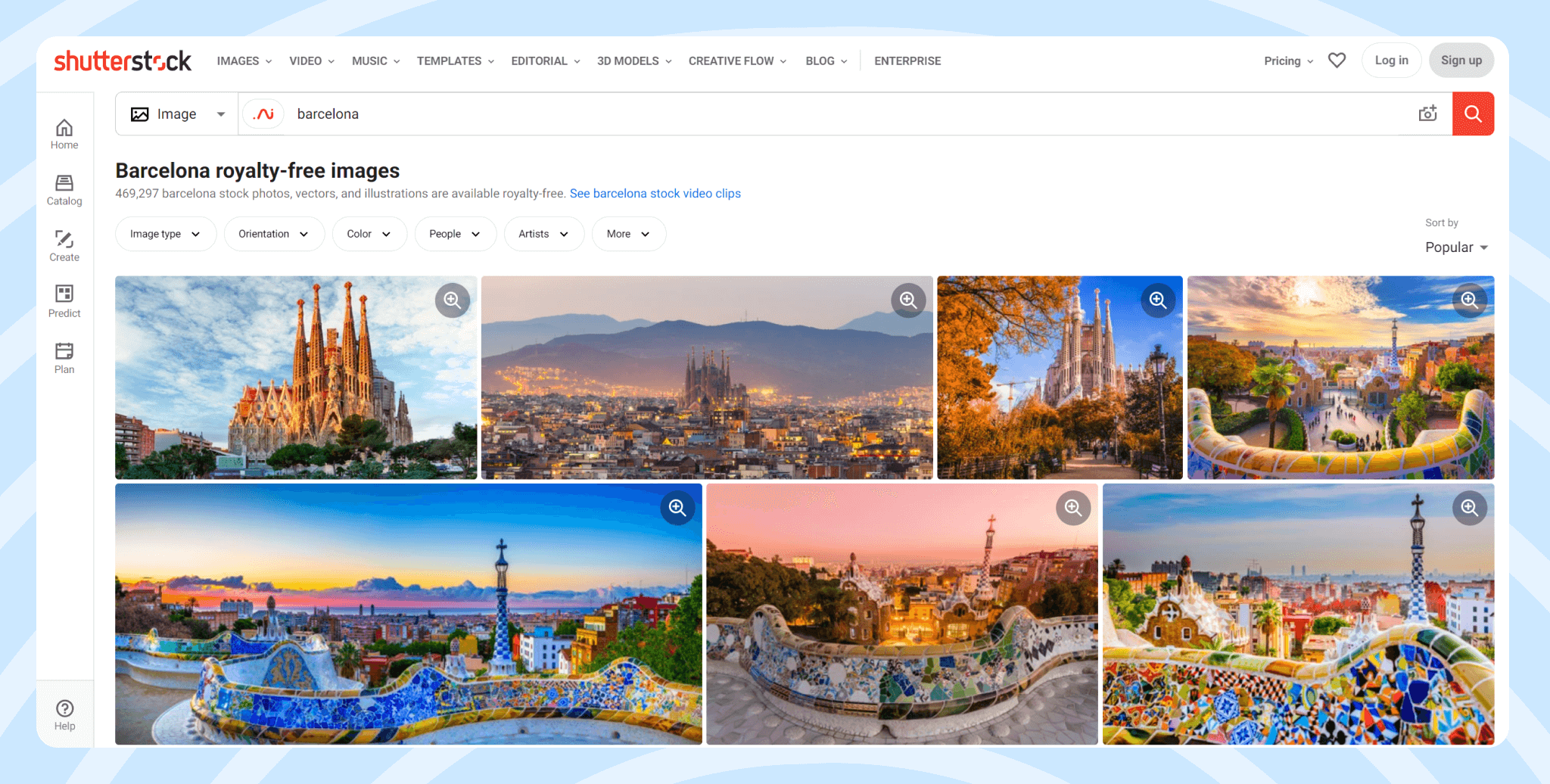This image is a high-resolution screenshot of a Shutterstock advertisement page focused on photography. The layout is landscape-oriented, approximately twice as wide as it is tall, and is framed against a gradient blue background adorned with subtle diagonal light blue lines, adding a stylish visual effect. Within this frame, a prominent white rectangular box with rounded edges hosts the main interface.

In the top left corner of the interface sits the Shutterstock logo, showcasing "shutter" in orange and "stock" in black, with the exception of a creatively designed orange "O" intersected by a diagonal white line. Adjacent to the logo, a navigation bar offers links and drop-down menus for various categories: Images, Video, Music, Templates, Editorial, 3D Models, Creative Flow, Blog, and Enterprise. To the right of the navigation bar, options for Pricing (with a drop-down menu), Favorites (marked by a heart logo), along with Login and Sign-Up buttons are neatly aligned.

Below the navigation bar, an interactive search box is present. Inside, "Barcelona" is pre-selected in the dropdown field dedicated to image categories. The search function is highlighted with an attractive orange search button featuring a white magnifying glass icon. Just beneath the search box, text indicates over 470,000 royalty-free images related to Barcelona.

The main content of the page displays a grid of stock photos, organized in two rows. The first row contains four images, while the second row presents three. These images are characterized by their vibrant, sharp, and colorful depictions of Barcelona, encapsulating the city's essence and vibrancy.